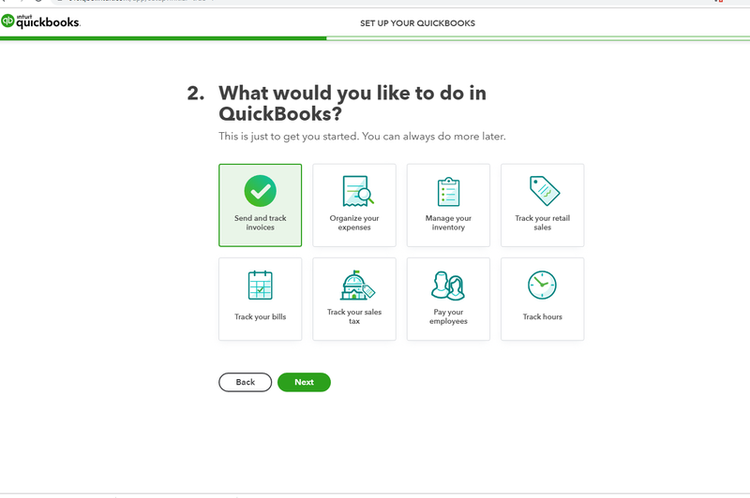The website screenshot captures the Intuit QuickBooks interface. At the top, a green progress bar stretches across, with its dark green-filled segment extending nearly to the center. Below the bar, bold text reads "2. What would you like to do in QuickBooks?" followed by lighter, thinner text stating, "This is just to get you started, you can always do more later."

The screen is divided into two rows of four boxes each. In the bottom left corner rests an oval white button labeled "Back," and adjacent to it, a green-filled oval button labeled "Next" in white.

In the first row of icons, from left to right:
1. A green circle contains a white check mark.
2. "Organize your expenses."
3. "Manage your inventory."
4. "Track your retail sales."

In the second row:
1. "Track your bills."
2. "Track your sales tax."
3. "Pay your employees."
4. "Track your hours."

The structured layout and clear navigation options aim to facilitate a streamlined user experience for QuickBooks newcomers.